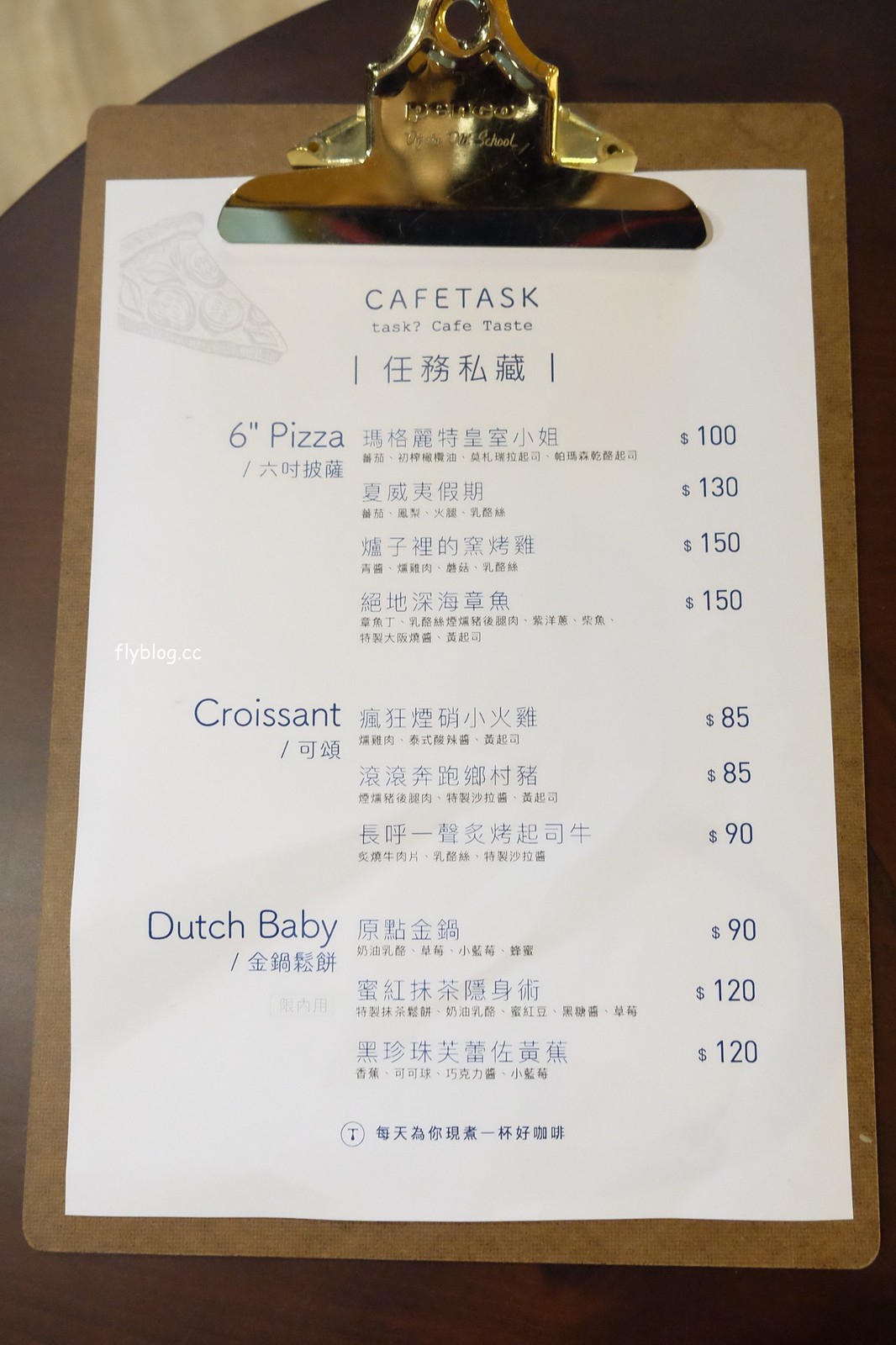The image is of a pizza restaurant menu titled "Cafe Task." The menu is printed on standard white printer paper and attached to a gold Penco clipboard, which bears some scratches and has slightly legible text under the brand name, possibly related to school. The clipboard itself is brown. The menu text is all in blue ink, with the word "Cafe Task" prominently displayed at the top, followed by text in an Asian language. Below this header, the menu lists items such as "6-inch pizza," "croissant," and "dutch baby," each accompanied by descriptions in the same Asian language. Prices for these items range from $85 to $150, situated to the right of each item. Along the left edge of the paper, there's a watermark reading "Flyblog.cc." The clipboard is positioned on a brown wooden table.